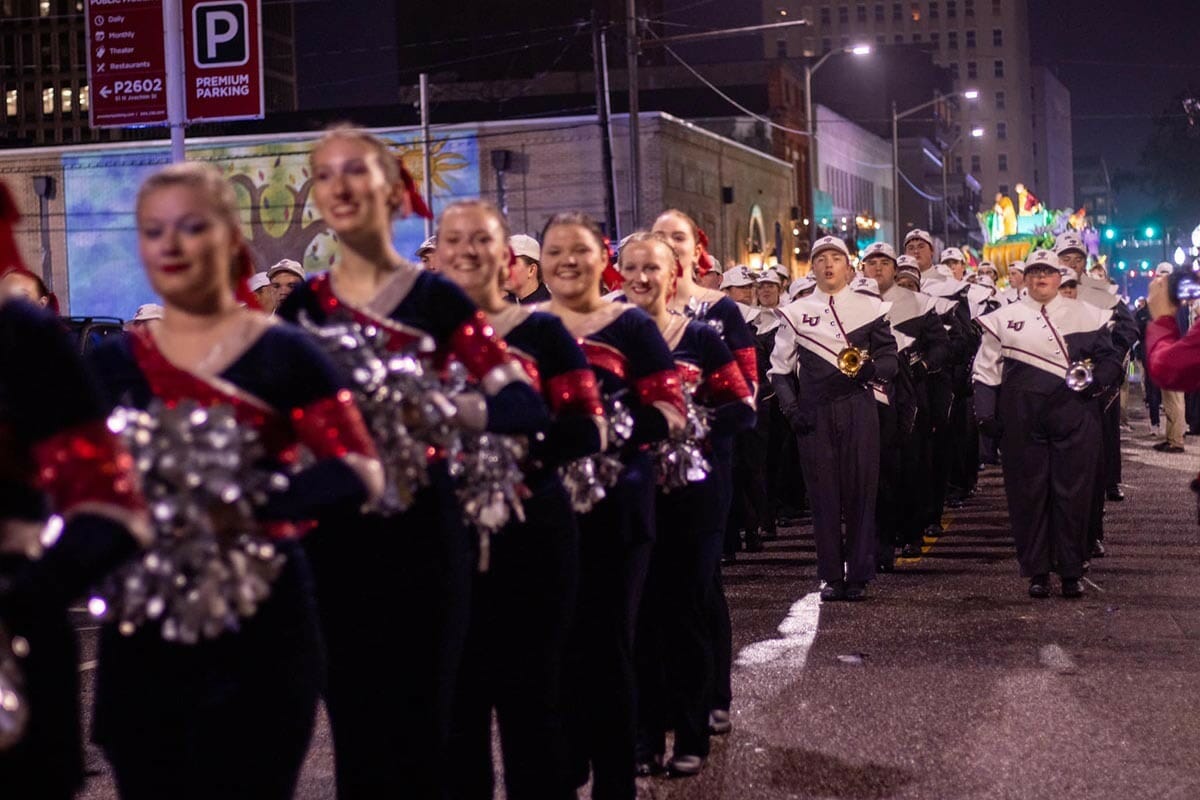In a nighttime downtown street parade, a row of young women stands at the front, dressed in striking black outfits with shiny red details on their arms. Each woman holds a glimmering silver pom-pom, and their hair is styled in ponytails adorned with red ribbons. They display radiant smiles as they perform. Behind them, several rows of men in marching band uniforms—white tops with black pants, accented by white shoulder straps, and white caps—hold circular musical instruments. The scene is set against the backdrop of city buildings and skyscrapers, with spectators visible on the right side, capturing the festive moment with photographs. A flagpole with a "P Premium Parking" banner adds to the downtown ambiance, confirming this lively event is taking place on the right side of the street.